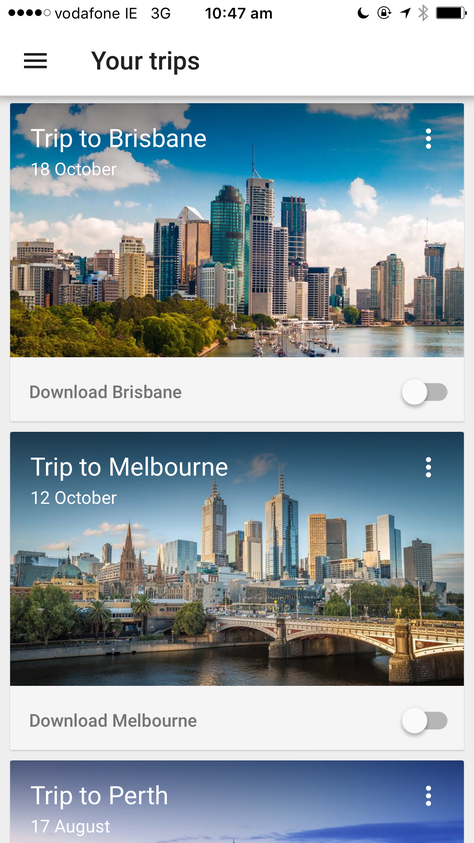The image is a screenshot taken from a mobile web browser. At the top, there are five horizontally aligned circles—four black and one white—indicating some form of progress or status. Next to the white circle, the text "Vodafone IE 3G" appears in black font. The top center displays the time as "10:47 AM." On the upper-right corner, there are various icons: a half crescent moon, a lock symbol with a circular arrow around it, an arrow pointing upwards to the right, a grayed-out Bluetooth icon, and a nearly full battery icon.

Below this top bar, there's a black hamburger menu icon (three horizontal lines) followed by the text "Your Trips." The page is divided into three main sections, each featuring a photograph and accompanying text.

The first section showcases an expansive city skyline featuring skyscrapers and large buildings under a partly cloudy sky with blue and white hues. In the foreground, there is a marina to the bottom right and a lush green forest to the bottom left. The overlay text in white reads "A Trip to Brisbane," with the date "18 October" beneath it. A gray banner at the bottom of this photo reads "Download Brisbane," accompanied by a toggle button that appears to be off.

The second section mirrors the first in layout but highlights Melbourne. The image features a city skyline with numerous skyscrapers, a bridge at the bottom right, and a river flowing nearby. The sky is again a blend of blue and partly cloudy conditions. The text states "A Trip to Melbourne," with the date "12 October" appearing at the top left of the image. Below, a gray banner reads "Download Melbourne," with an adjacent inactive toggle button.

The third section is partially cropped, showing mainly a blue sky. Text on the left side reads "Trip to Perth," with the date "17 August" in white letters below it.

Overall, the screenshot captures a neatly organized travel itinerary page with vivid cityscape images and associated trip details.